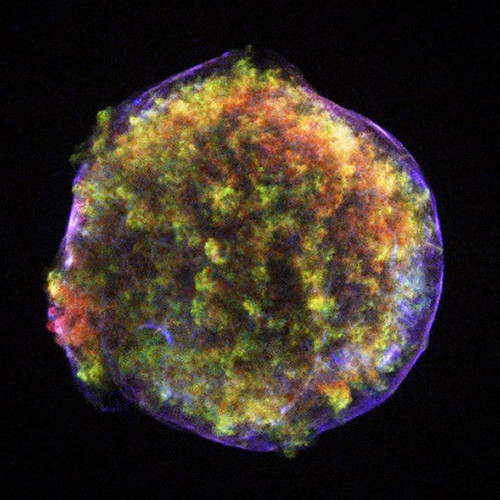The image, square in format, presents a central circular area set against a solid black background, creating a striking contrast. This central circle features a glowing purple rim that frames a complex, multi-colored interior. The variety of colors within the circle gives it a dynamic and organic appearance. Predominantly green at its core, it is interspersed with vibrant orange, red, and yellow hues, especially towards the outer edges. This composition could be interpreted in various ways: it might resemble a microscopic photograph of a bacterial culture in a petri dish, with the colors representing different stages of growth, or it might be an artistic abstraction depicting an aerial view of a densely forested area from high above, with green leaves mingling among those turning with the seasons.